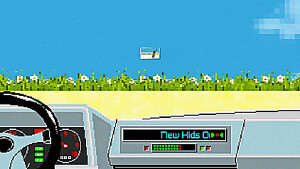This image showcases a computer-generated scene from the inside of an older model car, characterized by a large, boxy dashboard. The black steering wheel is prominently positioned, with a horn in its center. The dashboard features a variety of controls and gauges, including a miles-per-gallon gauge. The car's radio displays "New Kids On" in blue text, and the volume controls are highlighted in green.

Through the car's windshield, a tranquil beach scene unfolds. The cream-colored sand is dotted with computer-rendered plants adorned with daisy-like flowers. The background reveals a serene expanse of blue, which might be the sky or water. Additionally, a small, blue and white advertisement or sign is visible in the distance, adding an extra layer of detail to the scenic backdrop.